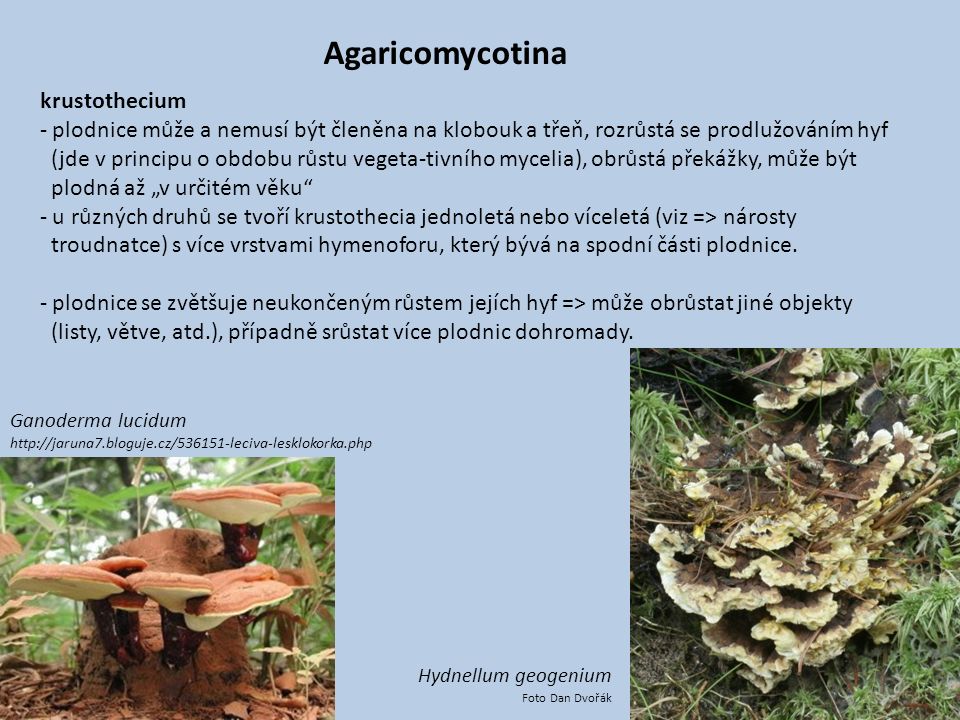The image depicts a PowerPoint presentation slide with a light blue background. The title at the top is "Agarico omekutina," followed by the word "chrysothecium" and three bullet points, all written in what appears to be Polish. In the bottom left corner, there's an image of mushrooms labeled "Ganoderma Lucidum" in italicized black letters. These mushrooms are attached to what looks like a red rock, with red, flat tops and white undersides, set against a backdrop of green leaves. In the bottom right corner, another set of mushrooms is labeled "Hydnelum geogen" in italicized black letters. These mushrooms appear brown with yellow edges and have a wavy, ruffled appearance, lying amidst some grass. The color palette includes blue, black, green, orange, brown, and white.